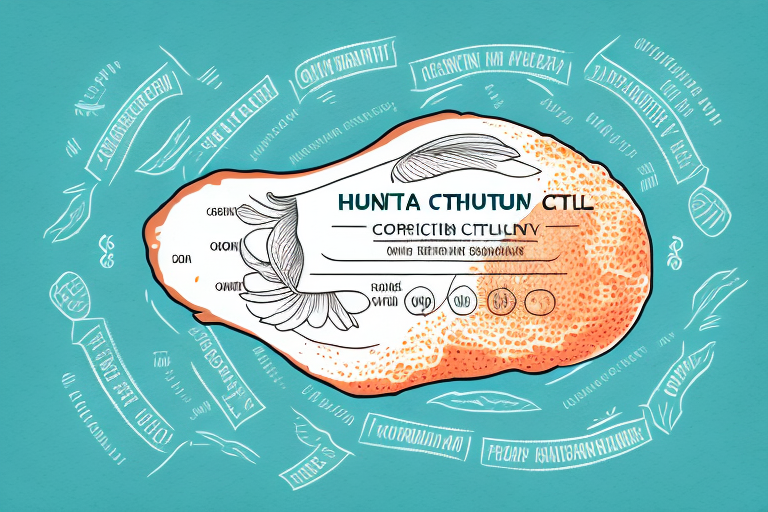The image features a predominantly teal background with a more blue-green hue and displays intricate details and text. At the center of the image, there is an oval, peanut-shaped figure with a light orange tint, framed by white banners or ribbons flowing around it. These banners contain white shapes and Cyrillic-like letters, often hard to decipher, written in dark, likely black, ink. Central text includes "Hunita Tuhatun" (or similar variations such as "Honita Tuhatun") and potentially "Steel Correction Facility," suggesting a tough-to-read or foreign script. Surrounding the central orange figure with a white blob overlay, there are illustrations resembling a fish or seashell, intermixed with leaves and other shapes. An additional note mentions a blue banner with white lettering reading "Trump Administration." The overall ambiance offers a hand-drawn sketch style with an intricate mix of shapes and lettering, blending a whimsical and slightly confusing array of linguistic elements.